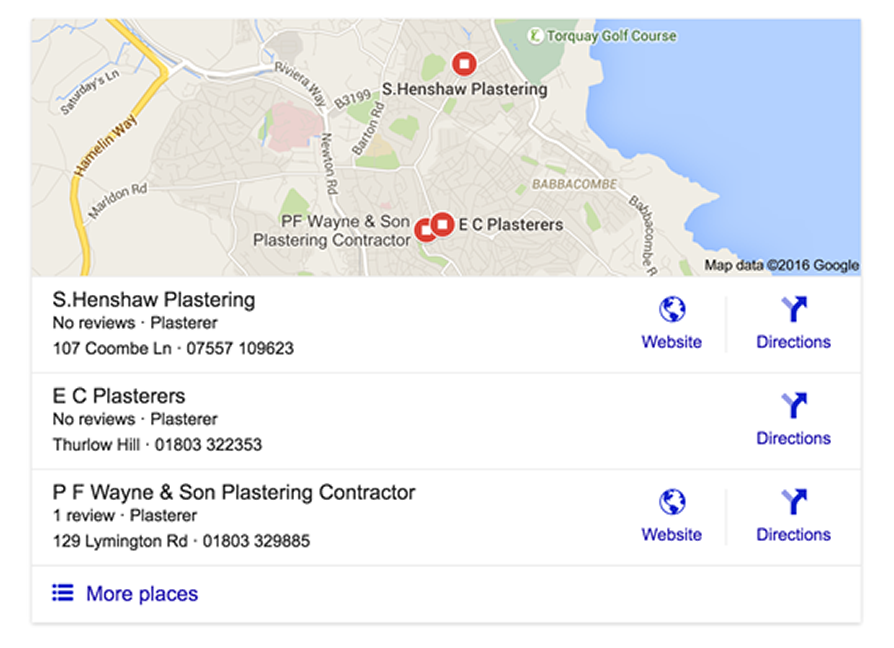This cropped screenshot appears to be a snippet from Google Maps search results, potentially displayed on the right-hand side of a search page. The search seems to pertain to plastering services, featuring three distinct plastering companies. The map, dated from 2016, hints that this information is slightly outdated. The search results showcase the following companies:

1. **S. Henshaw Plastering** - This listing includes the company's location, phone number, and information on Google reviews.
   
2. **EC Plasterers** - Similarly, this company’s basic contact details are displayed.
   
3. **PF Wayne and Son Plastering Contractor** - This entry also features relevant contact information.

Each company listing includes an option to visit their website (if available) and a 'Directions' button for navigation purposes. Additionally, there is a 'More places' button located at the bottom-left corner, allowing users to explore other plastering companies in the vicinity. Based on one of the city's names, "Babacombe," this search is likely conducted outside of the USA, possibly in a region like the UK.